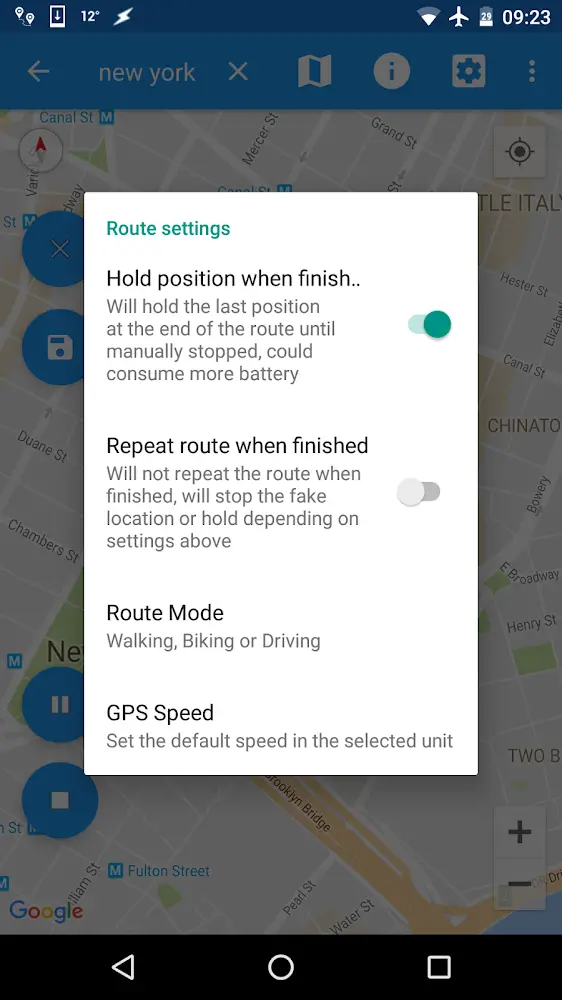The image depicts a cell phone screen with a semi-transparent gray overlay that partially obscures the background. In the upper right corner of the screen, the status bar displays various icons: a wireless connection symbol, an upward-pointing airplane icon, and a battery indicator showing '29'. The time displayed is 9:23 AM.

Below the status bar, a blue section reads "New York" and features an array of symbols, including an 'X' for closing, an 'i' enclosed in a circle for information, and a gear icon within a square, likely representing settings.

Most of the screen is occupied by a map, albeit difficult to discern due to the presence of a white pop-up overlay. Some streets are labeled, and four blue dots are visible, presumably marking specific locations, but their exact details are obscured by the pop-up. In the bottom-left corner of the map section, the word "Google" is subtly present.

At the very bottom of the screen, there is a black border that spans the width of the device, containing navigation icons: a triangle pointing left (back button), a circle (home button), and a square with a white border (recent apps button).

The prominent white pop-up on the screen is labeled "Route Settings" and provides various instructions and settings options, including:
- "Hold position when finished... Will hold the last position at the end of the route until manually stopped. Could consume more battery." This option is currently selected.
- "Repeat route when finished," which is not selected.
- "Route mode" offering choices for walking, biking, or driving.
- "GPS speed," allowing the default speed to be set in the selected unit.